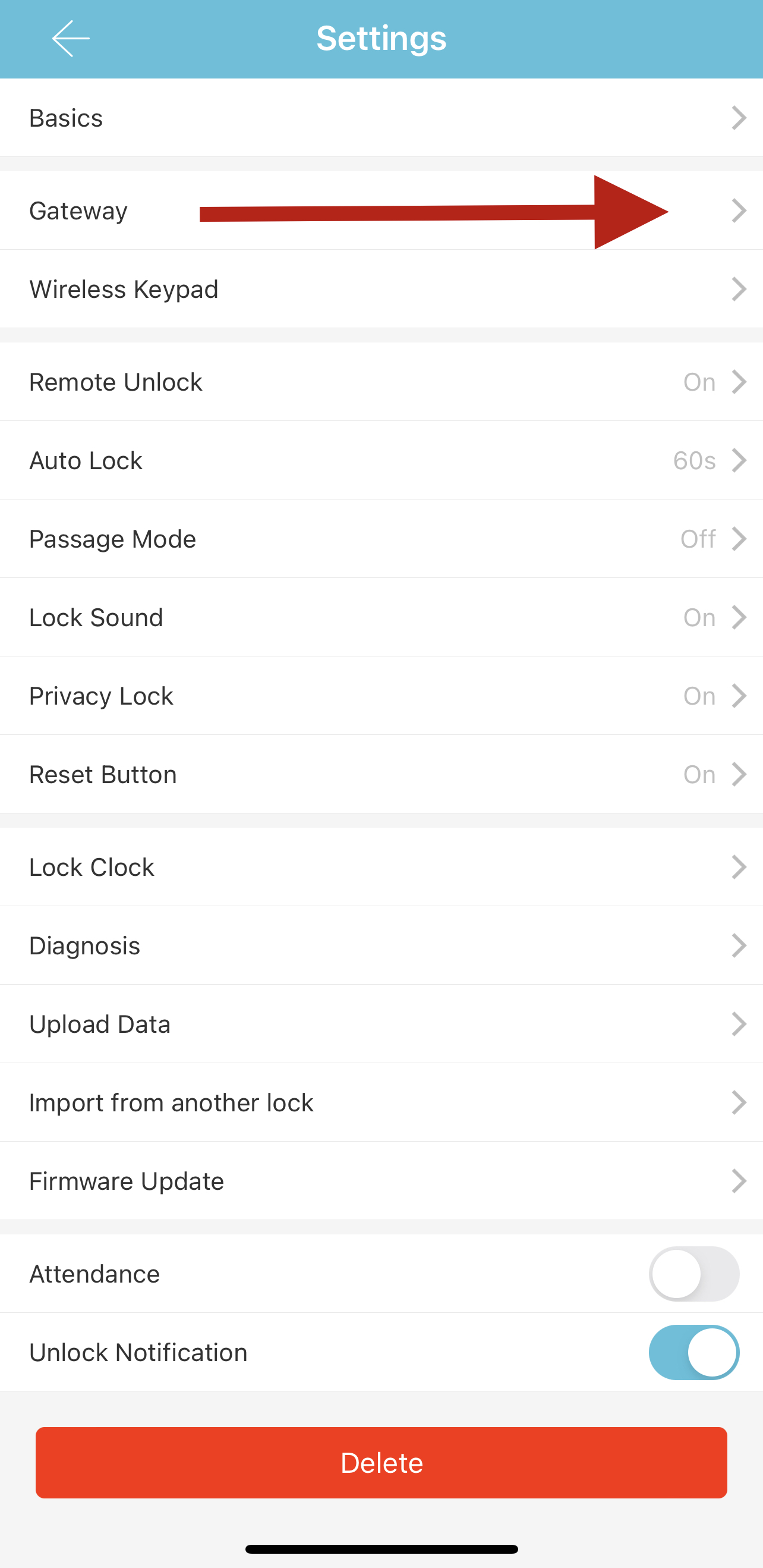The image showcases a settings page from an application running on a smartphone, displayed in a portrait orientation. Dominating the top of the screen is a light blue rectangular header with white text centered in it, which reads "Settings" with a white left-pointing arrow on the left side, suggesting a back navigation option.

Directly below this header is a series of settings options structured into distinct sections, all contained within white rectangular boxes with thin grey borders. The first section includes an option labeled "Basics," displayed with black text on the left and a right-pointing arrow on the right, indicating a clickable menu item. 

Following this, two more options are listed: "Gateway" and "Wireless Keypad." Notably, the word "Gateway" is accompanied by a red arrow pointing right towards the right-pointing arrow at the end of the line.

Next, a more comprehensive category appears, listing several configurations:
- Remote Unlock: On
- Auto Lock: 60 seconds
- Passage Mode: Off
- Lock Sound: On
- Privacy Lock: On
- Reset Button: On

Each setting displays its status or configuration detail adjacent to right-pointing arrows.

Further down, there are additional settings options which include:
- Lock Clock
- Diagnosis
- Upload Data
- Import from Another Lock
- Firmware Update
- Attendance
- Unlock Notification

The "Unlock Notification" option has a blue toggle switch set to 'On' on the right side.

Finally, at the bottom of the settings page is a prominent orange button with white text that reads "Delete," presumably for deleting all settings or the associated account or item.